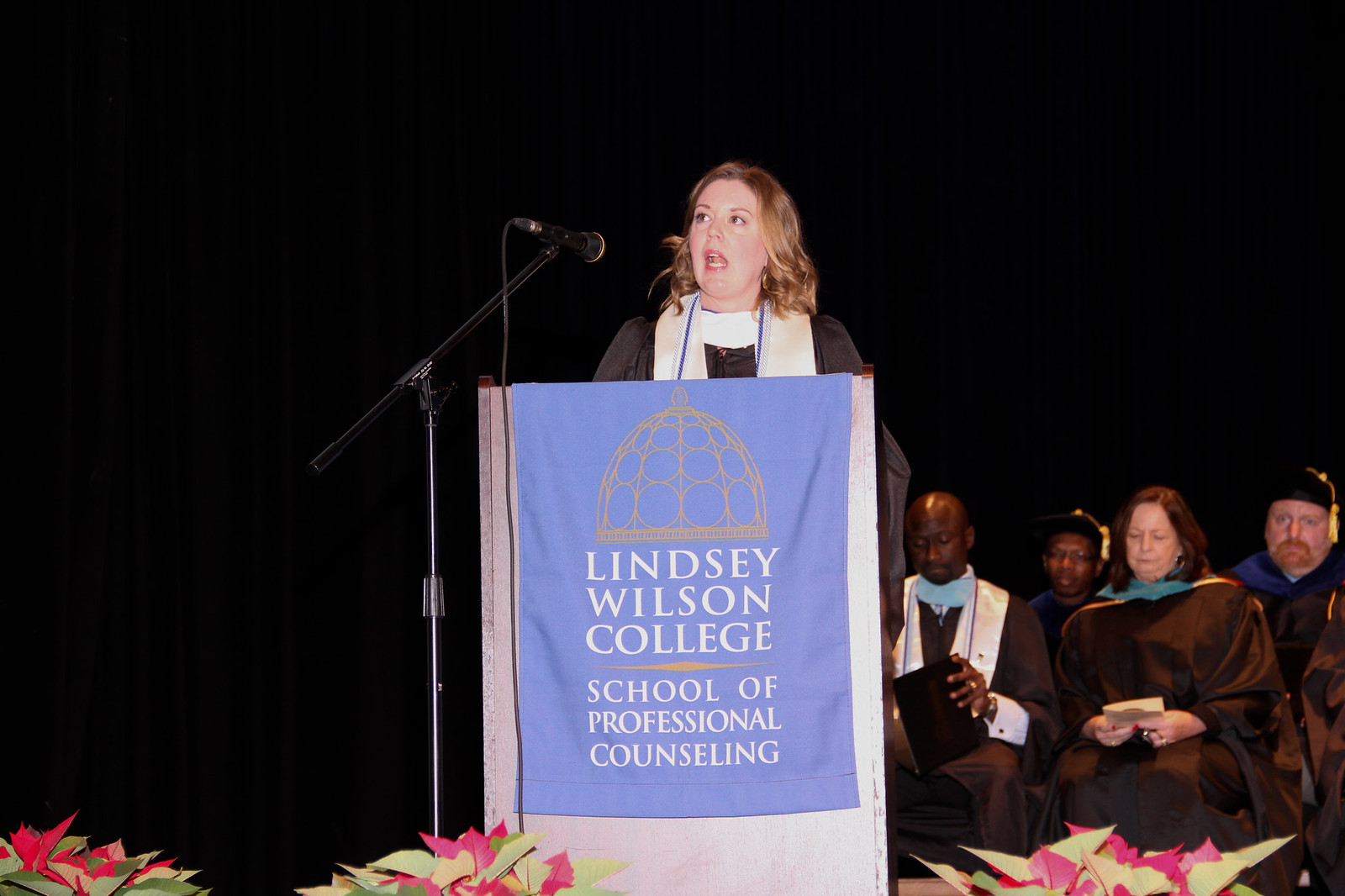In the image, a woman with long wavy brown hair is speaking into a wired microphone at a wooden podium, illuminated by light, suggesting possible flash photography. The podium features a blue banner with white text reading "Lindsay Wilson College, School of Professional Counseling." Above the text, there is a yellow emblem resembling a cage with circular designs. The woman is dressed in a black graduation gown and a long white sash. Behind her, the background is predominantly dark with a stage curtain of very dark brown. To her right, a group of seated individuals in black gowns and caps are visible; some are white, others black, and a few are reading papers, possibly practicing their speeches. Among them, some wear yellow sashes on their caps, while a man wears a white sash down the sides of his gown. The scene suggests a formal graduation ceremony.